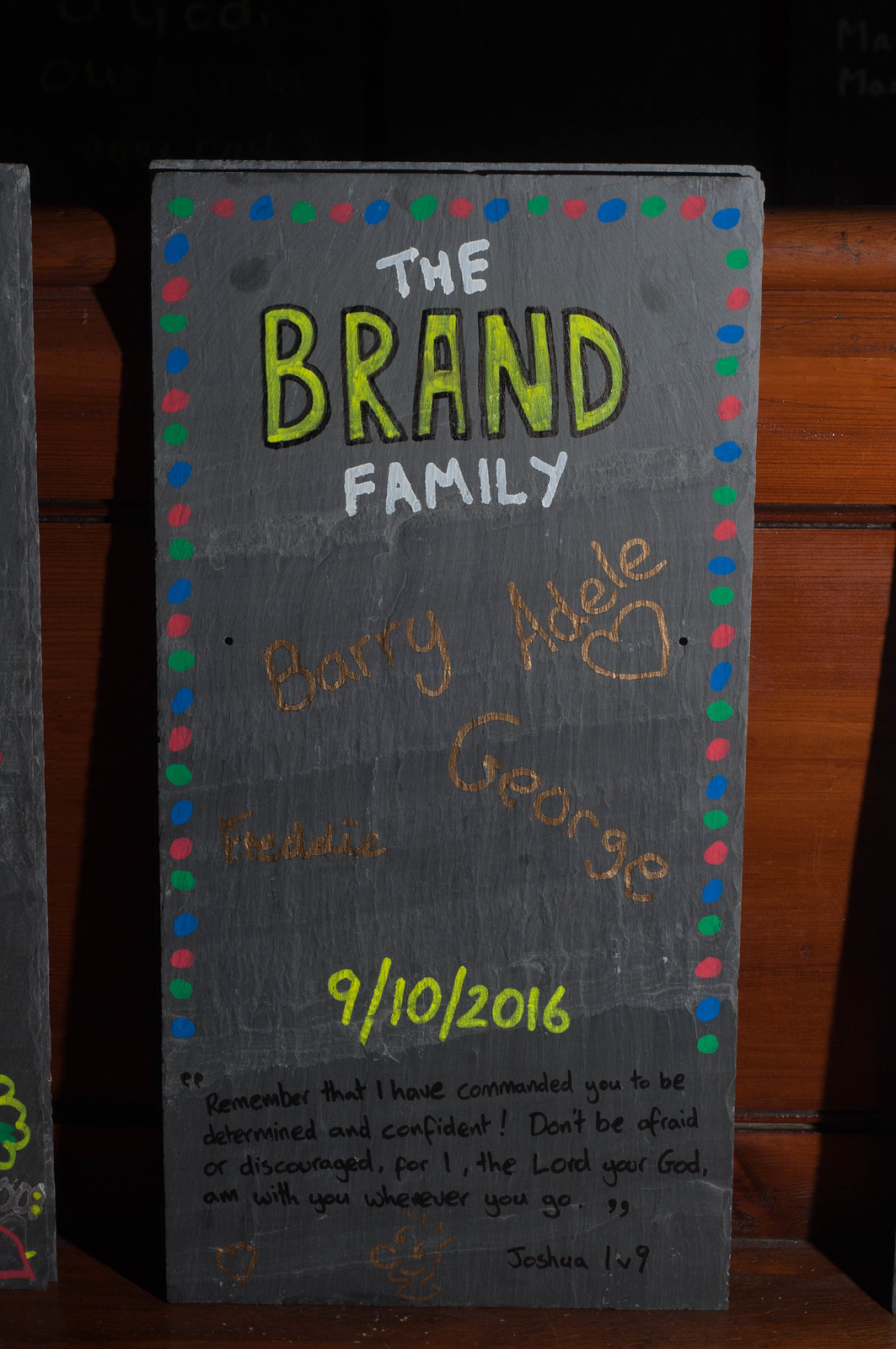A handmade, gray family sign with colorful green, blue, and red dot accents around the border is the focal point of the image. The sign, which leans against a wooden shelf in a dimly lit room, reads "The Brand Family" in prominent yellow letters at the top. Below this are the names "Barry," "Adele" (with a heart next to it), "George," and "Freddie," followed by the date "9/10/2016" in yellow. Beneath these details, a biblical quote from Joshua 1:9 is inscribed in black: "Remember that I have commanded you to be determined and confident. Don't be afraid or discouraged. For I, the Lord, your God, am with you wherever you go." The image also shows another object partially visible off to the left. The overall style of the sign gives it an artistic, heartfelt appearance, further accentuated by its placement in the home's cozy, wooden interior.